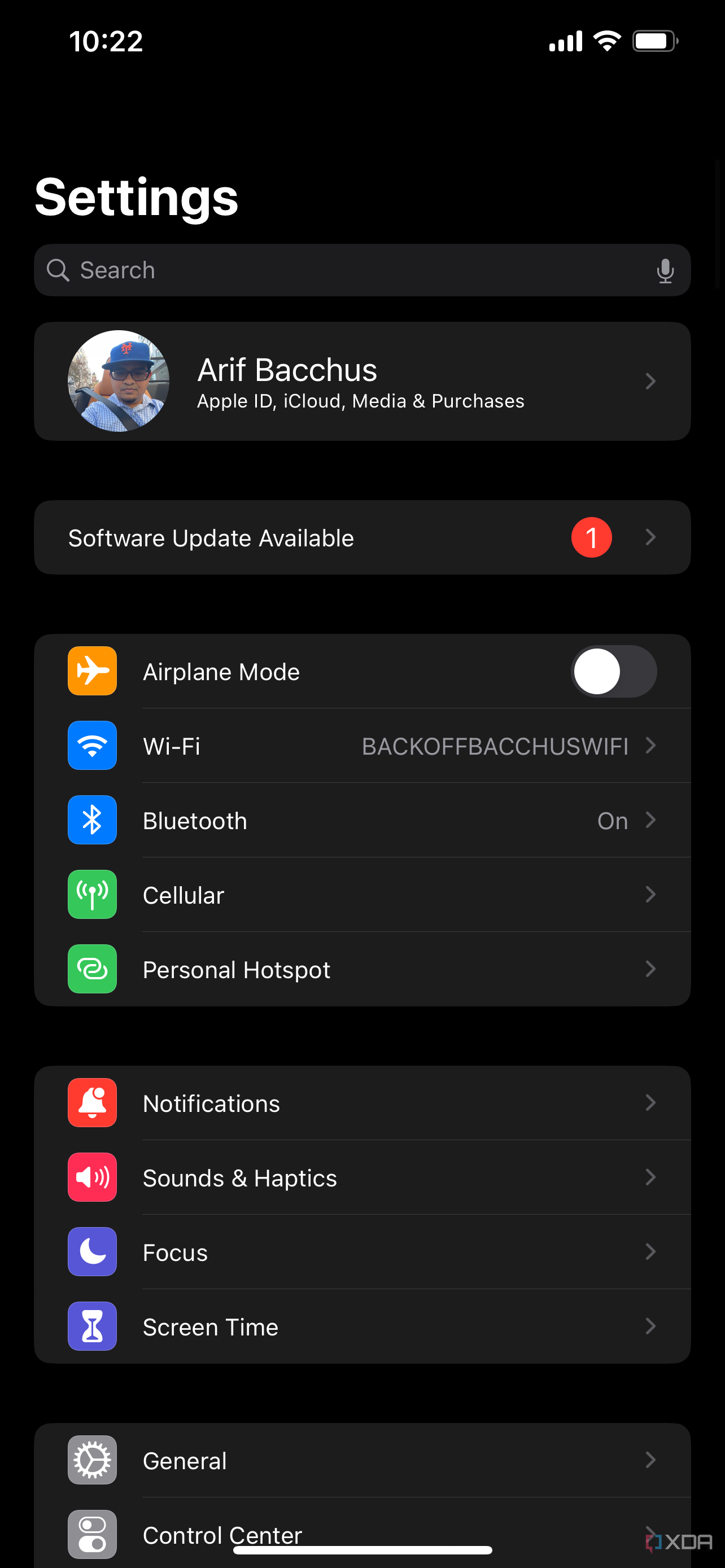Screenshot of a smartphone's settings menu, taken at 10:22 AM. At the top of the screen is a profile picture of a man who appears to be approximately 27 years old. He is wearing a blue hat and glasses, and he looks Hispanic. The photo shows him inside a vehicle, secured by a seatbelt. His name is displayed as Aerith Bacchus. Below his name, there are options for managing the Apple ID, iCloud, and media and purchases. A notification indicates that a software update is available.

The settings options visible include:
- Airplane Mode
- Wi-Fi: The current network name is "Back Off."
- Bluetooth: Currently turned on
- Cellular options
- Personal Hotspot
- Notifications
- Sounds & Haptics
- Focus settings
- Screen Time, with an icon resembling an hourglass
- General settings
- Control Center